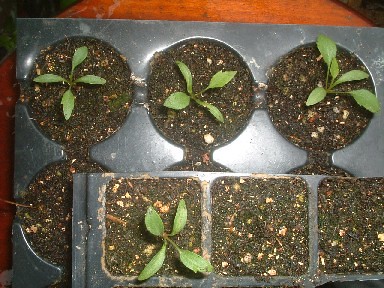The image, captured from an aerial viewpoint, showcases two distinct planters made of black hard plastic on a medium brown round wooden surface, set against a dark background. The first planter, reminiscent of a cupcake pan, features six circular openings arranged with three at the top and three at the bottom. The top three of these circular openings, along with parts of the first and last of the bottom row, are visible and filled with dark brown dirt speckled with white pebbles or rocks. Emerging from these openings are tiny green seedlings, each with four leaves.

Partially obscuring the lower row of the first planter is a second rectangular planter, which appears to be slightly raised or positioned on top of the circular one. This rectangular planter contains three square sections, each similarly filled with dirt and pebbles, and also hosts small four-leafed seedlings. Only one section in the foreground of this rectangular planter is planted. The overall arrangement and overlapping of the planters create a layered and orderly display of nascent plant life.